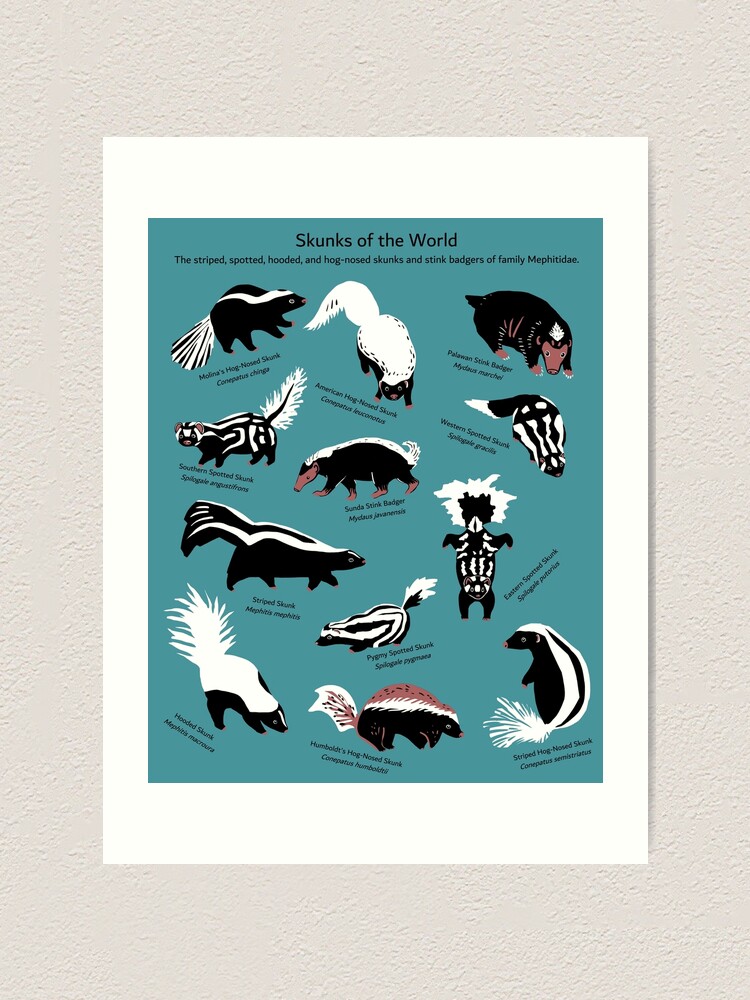The image appears to be a framed educational illustration titled "Skunks of the World." Set against a green background and bordered by a white frame, the poster is displayed on a slightly grayish-brown background, reminiscent of a wall. The text, all in black, reads "Skunks of the World" and further specifies, "The striped, spotted, hooded, and long-nosed skunks and stink badgers of family Mephitidae."

The illustration showcases 12 different skunks and stink badgers, each displaying unique white and black markings, with some also featuring reddish-brown hues. The animals are arranged centrally in horizontal and vertical rows. Each skunk is labeled with both common and Latin names, although the text is too small to read clearly.

Noteworthy variations include:
1. The typical American skunk with a white stripe.
2. A skunk with white fur on top and dark fur underneath.
3. A mole-like skunk with a stubby tail.
4. A black skunk with white stripes and a bushy white tail.
5. A black skunk with a long nose and a white stripe down its back.
6. A skunk with a distinctive white fuzzy head.
7. A black skunk with double white stripes down each side of its body.
8. A skunk with a red top, followed by a white band, and black underneath.

The illustration is not only visually appealing but also educational, aimed at providing detailed insights into the diverse family of skunks and stink badgers.